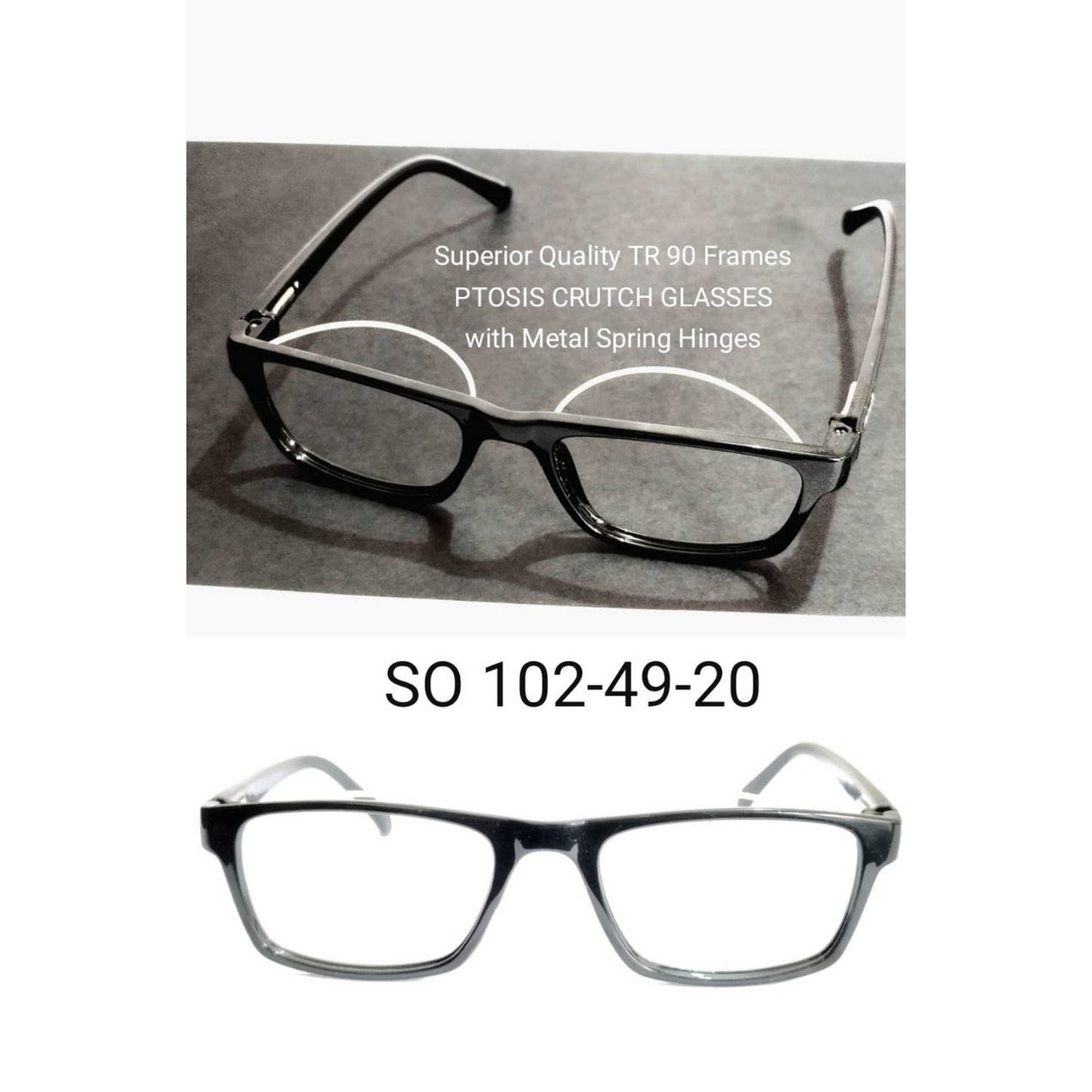This photograph is divided into two panels, one on top of the other. The top panel features a sleek pair of eyeglasses set against a gray background. Above these glasses, white text reads "Superior Quality TR90 Frames, Pitosis Crutch Glasses with Metal Spring Hinges." The frames themselves are described as dark steel gray metallic, with a noticeable white line arching from the back of the frames. The legs of the glasses are fully open, displayed for clarity. The bottom panel contrasts with its white background, displaying a different pair of eyeglass frames in a front-facing view, appearing more typical and less distinct compared to the top frames. In black letters above the second pair, the designation "SO102-49-20" is clearly shown. Both pairs of glasses seem to share a similar design, with the top pair emphasized for its superior quality and distinct features.